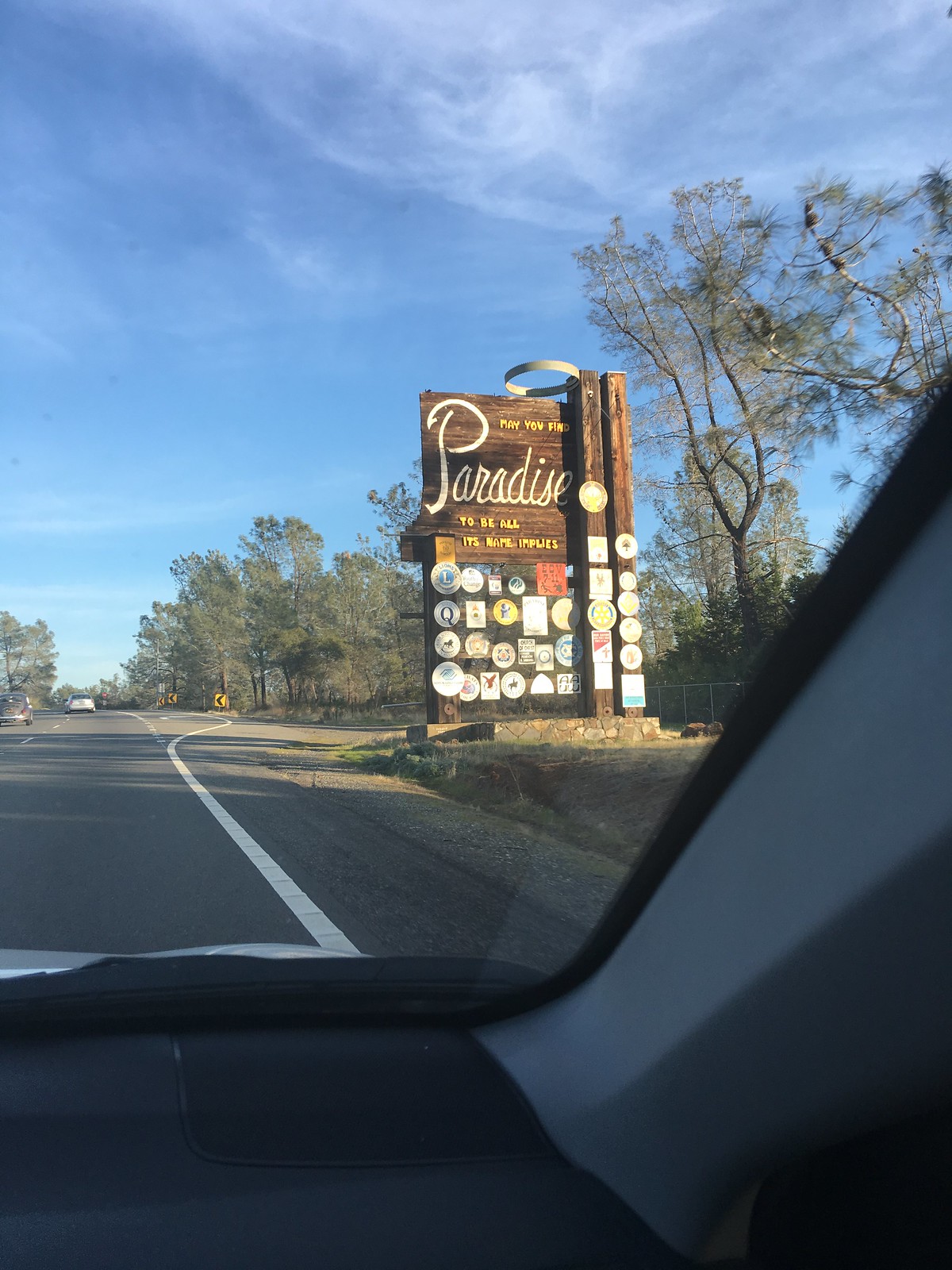A photograph taken from the passenger seat inside a car, capturing both the windshield and a portion of the car's interior, including a glimpse of the dashboard. The image focuses on a rustic, rectangular wooden sign with white script that reads "Paradise." Beneath this welcoming script, an inscription says, "May you find paradise to be all its name implies." The bottom part of the sign features several logos, likely representing local businesses or city councils, although the logos are indistinct in the image. The scene is set on a well-maintained asphalt road with a solid white line marking the right edge, suggesting that the location is either an entrance or exit to a place called Paradise. The sky above is clear and vibrant blue, adding to the idyllic atmosphere. Two other cars are visible ahead on the road, adding to the sense of a journey toward or away from this charmingly named locale.